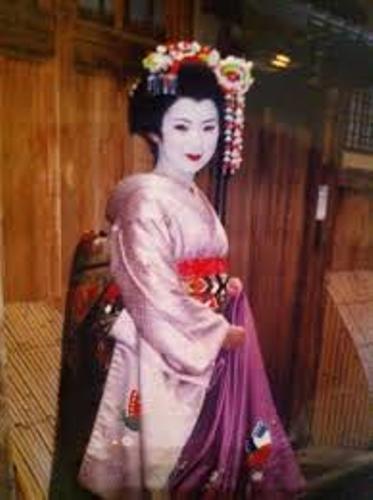The image features an Asian woman dressed in traditional geisha attire, standing inside a room with brown wooden panel walls and a matching floor. Her face is painted a striking powdery white, complemented by vivid red lipstick and a subtle, soft smile. Her black hair is styled neatly, adorned with a decorative headpiece featuring flowers in yellow, red, pink, and white, some of which delicately dangle on the left side of her face. She wears an elegant, light pink kimono made of shiny satin silk. The kimono, secured by a detailed red sash with black and white accents just below her bosom, extends into a magenta or bright purple skirt with intricate white and red designs. The woman stands with her arms by her sides, holding a piece of the purple satin fabric, and gazes directly at the camera, showcasing her beautiful, traditional ensemble.